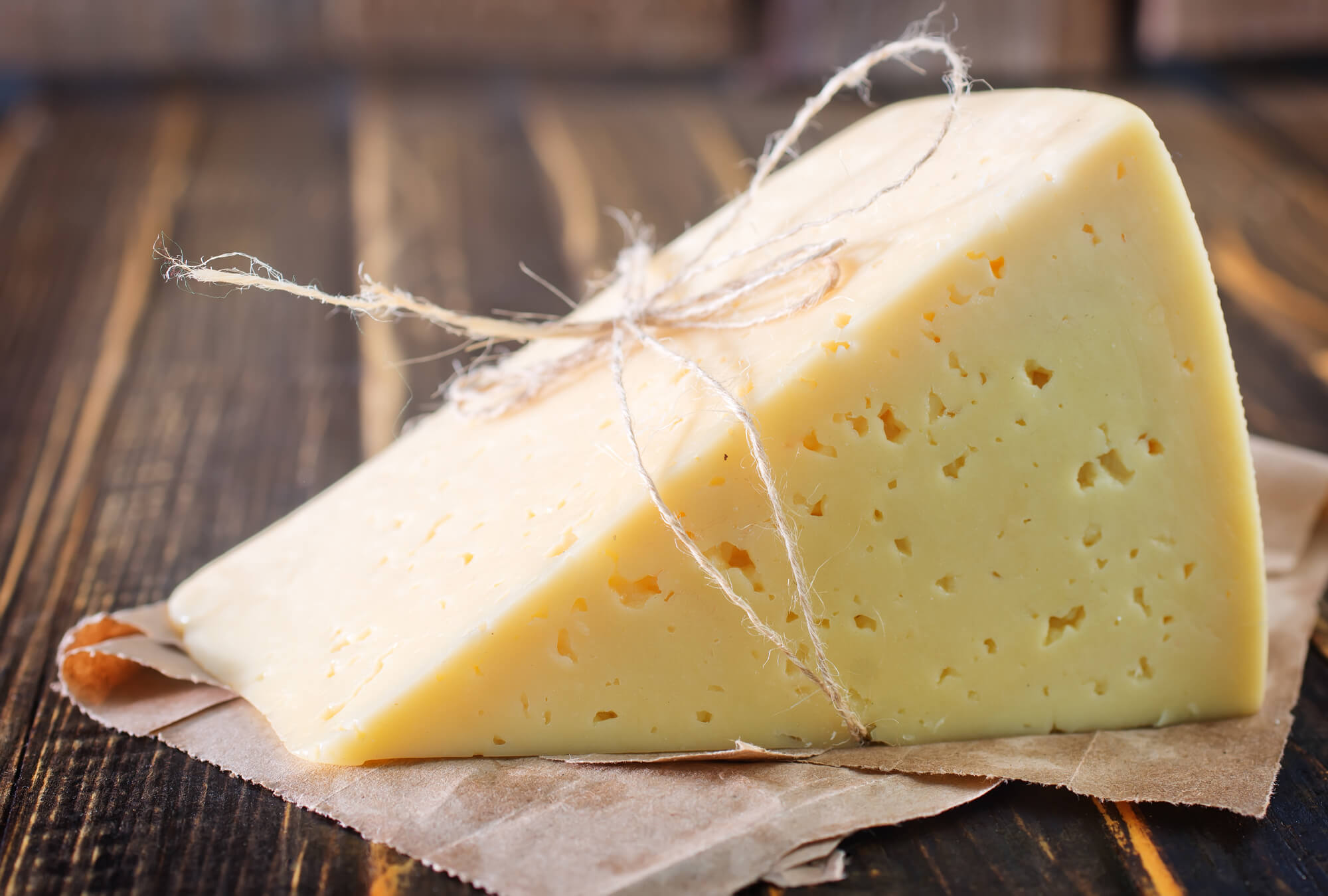This color photograph captures a detailed scene featuring a centrally placed wedge of cheese. The cheese, light yellow and dotted with small holes, is horizontally positioned with its sharper edge to the left and the larger side to the right. It is has a piece of brown twine tied around its middle, adorned with a bow. Resting underneath the cheese is a piece of greasy parchment paper, which soaks up the oils from the cheese. The entire scene is set on a dark walnut wooden table, characterized by subtle lighter stripes running through it. The light source originates from the left side of the image, illuminating the top of the cheese and casting a slight shadow on the side facing the camera. The combination of the table's texture, the greasy parchment, and the detailed cheese creates a rustic and appetizing atmosphere.